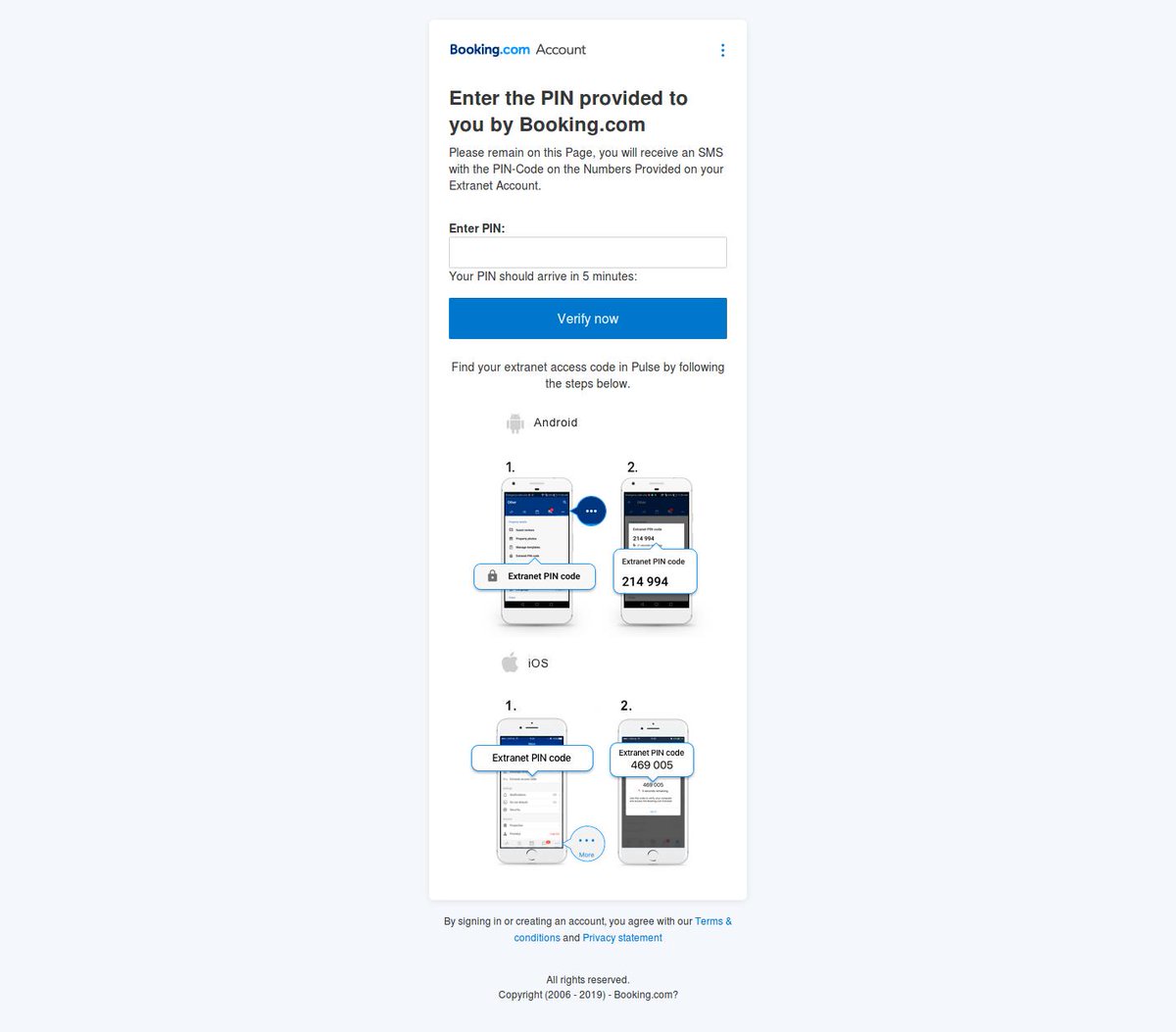The image displays a screenshot from the app version of Booking.com, specifically a page related to account verification. At the top left corner, 'Booking.com Account' is written in blue. Just below, in black text against a white background, instructions read: "Enter the PIN provided to you by Booking.com. Please remain on this page. You will receive an SMS with the PIN code sent to the numbers provided on your Extranet account."

Below these instructions is a box where users can enter the PIN, accompanied by a note stating, "Your PIN should arrive in five minutes." Adjacent to this box is a blue button labeled 'Verify Now.'

Further down, the page offers guidance on locating the Extranet access code in the PULT system. This section includes illustrative images of smartphones to depict the steps. At the top, there are two steps shown for Android devices: 

1. Getting the Extranet PIN code.
2. Entering the PIN code.

Similarly, for iOS devices, the instructions are displayed with images of phones labeled under 'Extranet PIN code' for both steps. The visuals aid users in understanding the process of entering their Extranet PIN code effectively.